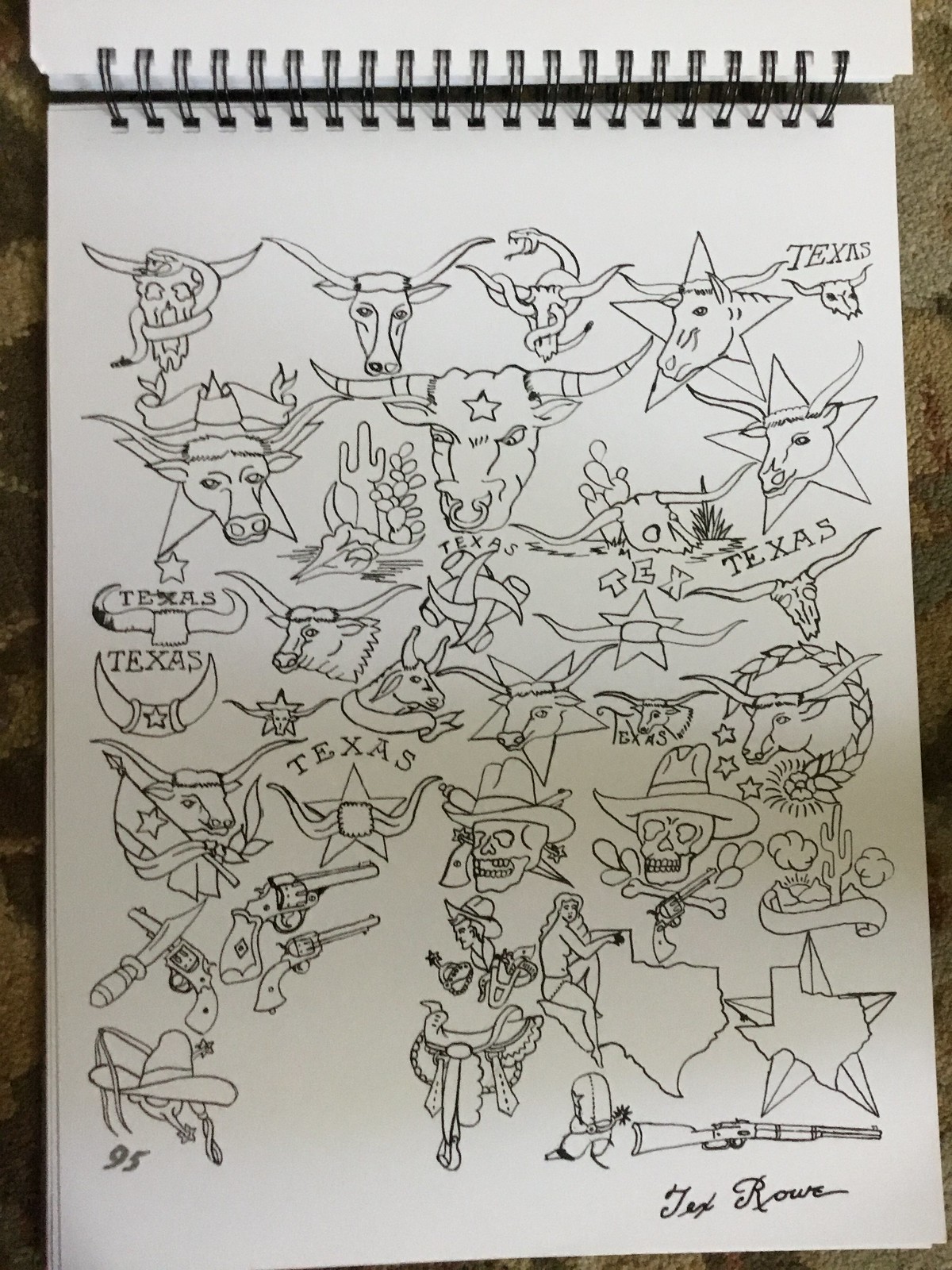This photo, taken from above, showcases an artist's sketchbook open on a beige tablecloth, with a spiral binding along the top edge. The white paper is densely covered in intricate black ink doodles featuring Western-themed imagery. Prominently displayed are multiple Texas steer skulls, some adorned with items such as a snake or placed inside a wreath. One skull is overlaid with a star, while another has "Texas" written above it. There are also several human skulls wearing cowboy hats, crossbones, and a notable sombrero marked with '95'. Some other key elements include cowboy boots with spurs, a Western saddle, revolvers, knives, a large rifle, and depictions of the state of Texas, including one centered in a star. At the bottom of the page, the artist has signed off with "Tex Rowe." This rich, detailed collection of drawings vividly captures the essence of Western iconography.